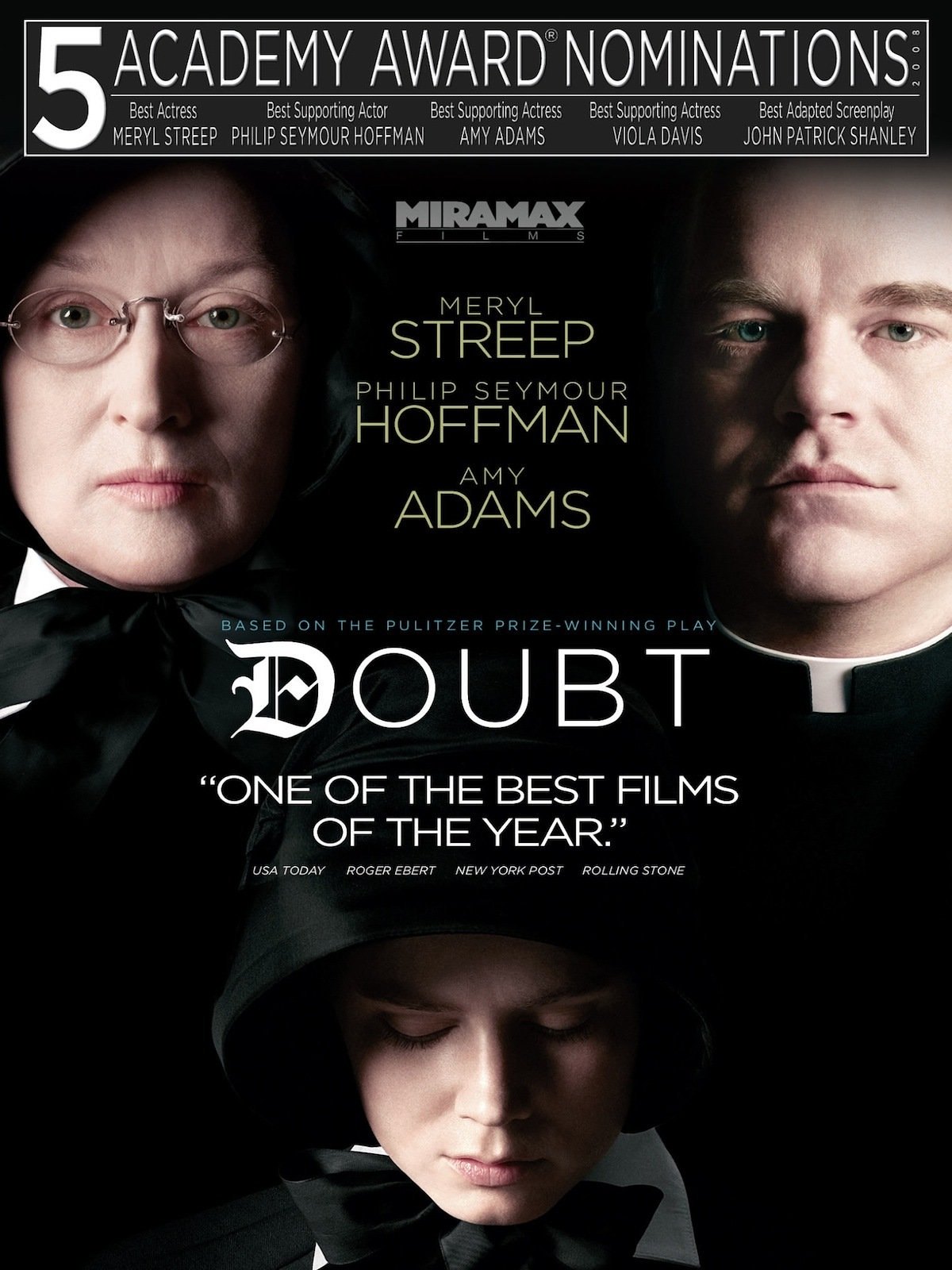This image is a movie poster for the film *Doubt*, prominently showcasing its five Academy Award nominations. Set against a very black background, the poster features three characters' faces: Meryl Streep on the left, Philip Seymour Hoffman on the right, and Amy Adams at the bottom. Both Streep and Adams are dressed as nuns, with Streep wearing glasses and a habit, and Adams looking downcast with a hood. Hoffman is portrayed as a priest, clad in a black shirt with a white collar. The poster's top features white text declaring the five Academy Award nominations, and below it, yellow text lists the main actors—Meryl Streep, Philip Seymour Hoffman, and Amy Adams. The title of the film, *Doubt*, is displayed in bold white letters along with the tagline, "One of the best films of the year." The poster also includes a tag for Miramax Films, the producer of the movie.